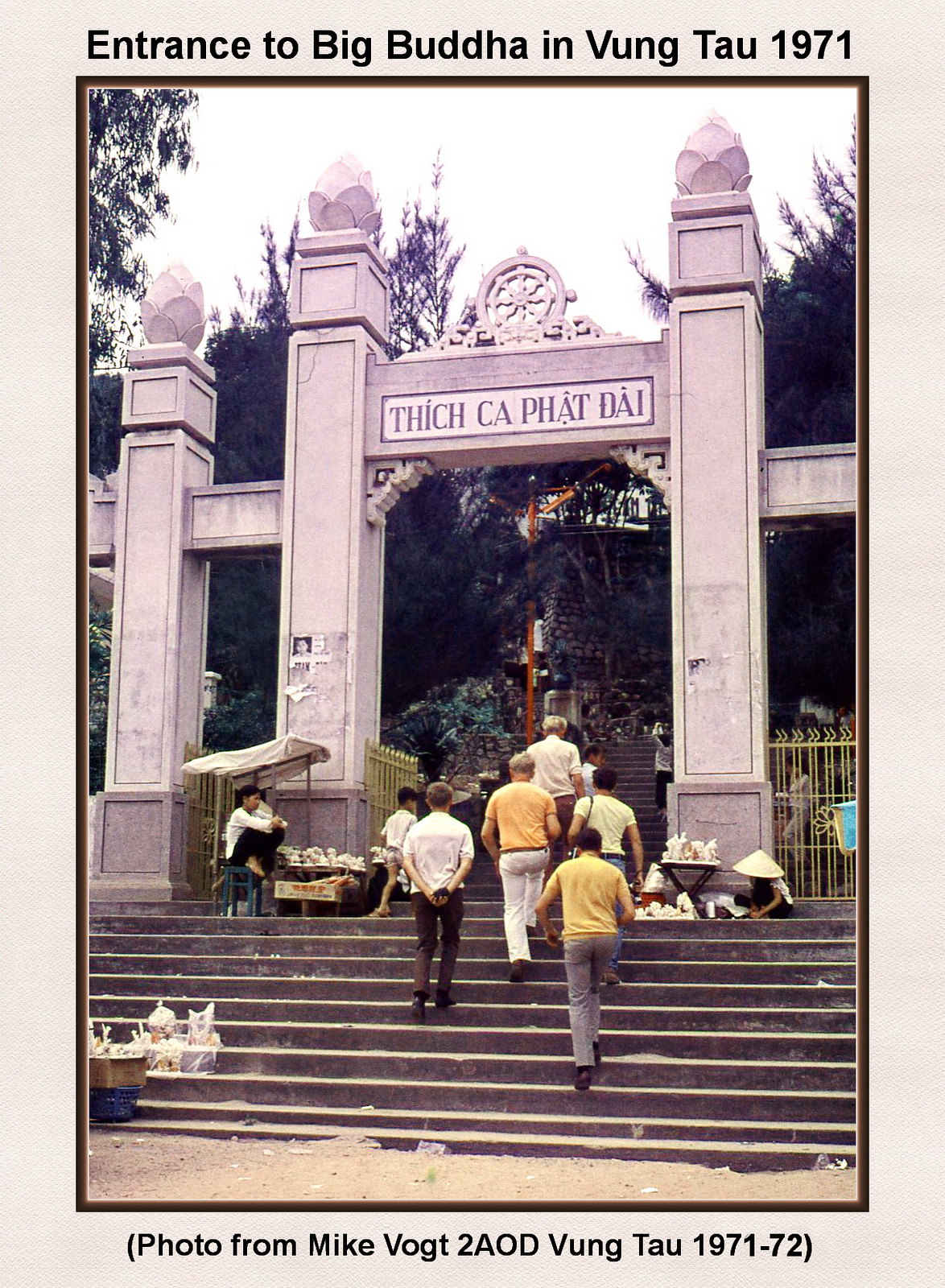This vintage photograph depicts an entrance adorned with large stone pillars leading up to an important site, identified as the "Entrance to Big Buddha in Vung Tau 1971" as indicated by black text at the top of the image. The entrance features an archway with an engraved sign that reads "Thick Ka Phat Dai." Below the archway, stairs ascend, bustling with people walking up and down. Some individuals are seen sitting on the steps, while vendors flanking either side sell their wares from small tables. The scene is outdoors with a backdrop of a white sky, glimpses of trees, and a brass or gold-colored gate. Two buckets are visible on the ground, adding to the worldly atmosphere captured in this historical image. At the bottom, in parenthesis, it states: "(Photo from Mike Vogt to AOD Vung Tau 1971-72)."